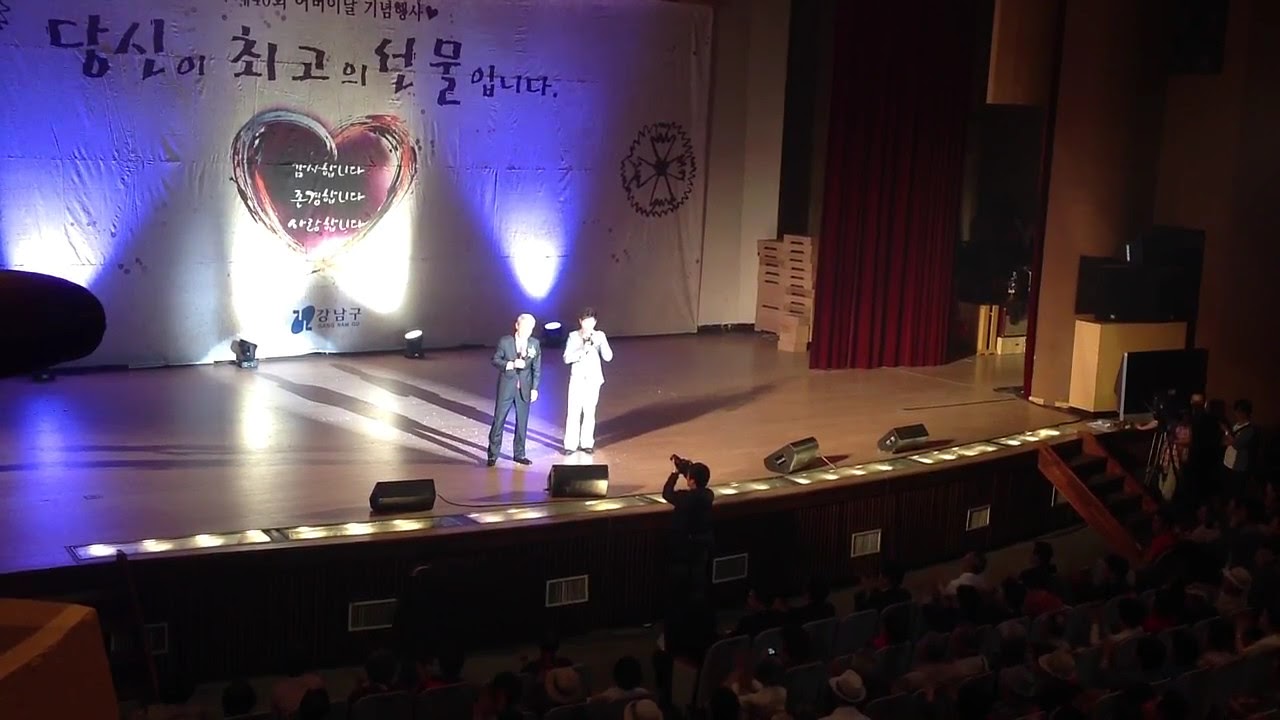This photograph captures a dynamic scene inside a large indoor auditorium from the vantage point of an audience member sitting toward the left side, looking toward the far right corner of the stage. The stage is brightly lit, with powerful spotlights illuminating two men standing between the backdrop and the apron. One man is dressed in a black jacket and pants, while the other wears a white jacket and pants, and both hold microphones. The backdrop features a heart symbol with Korean text inside and surrounding it. To the right edge of the stage, red curtains frame the scene, complemented by visible speakers and some stairs leading up to the stage. Below, a cameraman is positioned against the stage apron, capturing the moment. The audience area is filled with seated spectators, with some standing and clapping, adding to the vibrant atmosphere of the event.